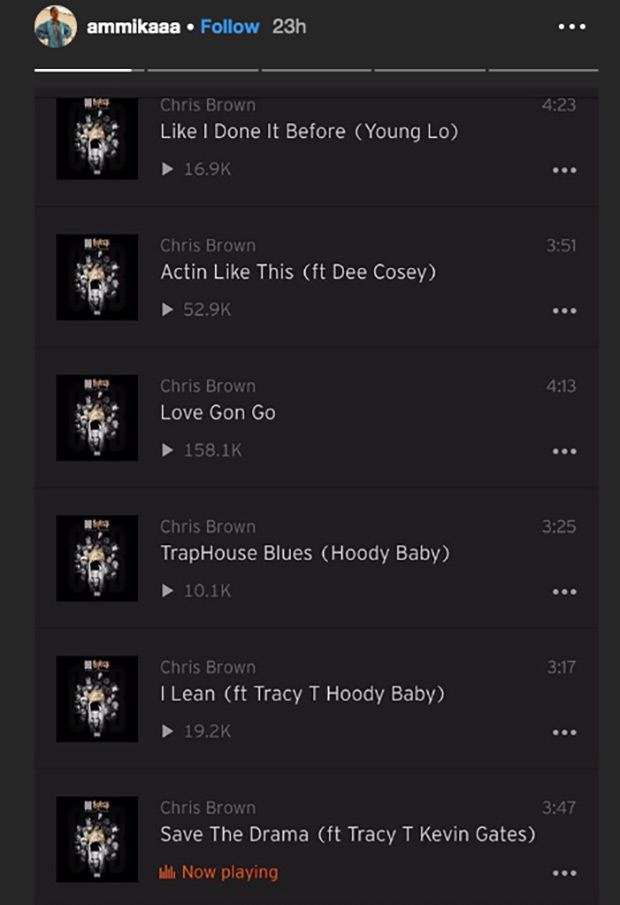This Instagram story, posted by user "AMMIKAAA" and marked with a grey "23H" timestamp, features a playlist of six tracks, all showcasing the same album cover art—a black square adorned with white dots and lighting effects at the center. "AMMIKAAA" is displayed in white text, with a profile picture to the left and a blue "Follow" button to the right. In the top right corner, there are three vertically aligned dots indicating more options.

The story consists of five segments, as shown by the five dashed lines at the top; the first is currently in focus, highlighted in white. Listed below are the six tracks, all by Chris Brown, featuring various artists:

1. "Like I Done It Before" featuring Yung Lo – 4:23
2. "Acting Like This" featuring Dee Cozy – 3:51
3. "Love Gone Go" – 4:13
4. "Trap House Blues" featuring Hoodie Baby – 3:25
5. "Eileen" featuring Tracy and Hoodie Baby – 3:17
6. "Save the Drama" featuring Tracy and Kevin Gates – 3:47 (currently playing, indicated by orange text)

The entire story is set against a black background, enhancing the visual focus on the text and album artwork.